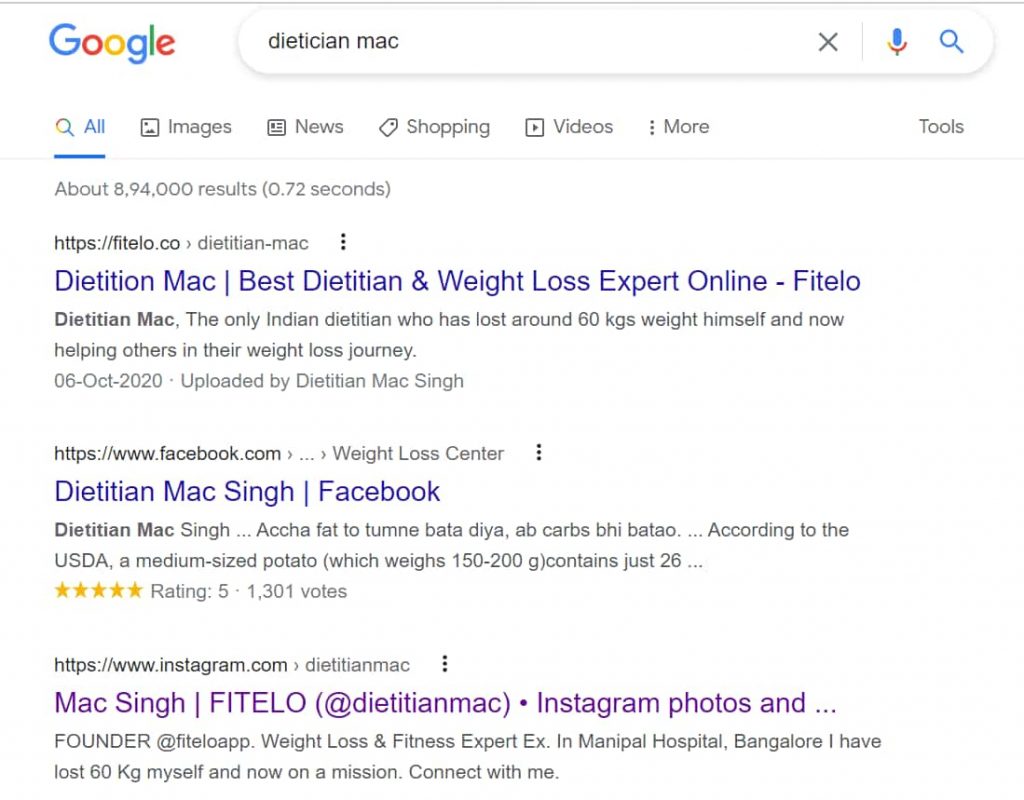Here's a detailed and cleaned-up caption for the provided image description: 

---

The image showcases a Google search results page. In the upper left corner, the familiar, multicolored Google logo is prominently displayed, consisting of a blue 'G', red 'o', yellow 'o', blue 'g', green 'l', and red 'e'. The search query entered is "Dietitian Mac". Below the search bar, there are typical Google search categories such as "All", "Images", "News", "Shopping", "Videos", "More", and "Tools".

The search results include a variety of links and descriptions. At the top of the results is a link to "Dietitian Mac". It is followed by descriptions including, but not limited to: "Best Dietitian Weight Loss Experts Online", "Philly TLAO Dietitian Mac", and mentions of being the only Indian dietitian to have navigated through a significant 16-week weight-loss journey, now aiding others in their weight-loss aspirations.

Next in the results is a Facebook link to "Dietitian Mac Singh". This profile features information like "IQFAT", an impeccable five-star rating, and lists Indian names such as "Chitturnabhata Bhattaraya" and "A. B. Gohan".

Further down the page is an Instagram link to "Dietitian Mac", a profile by "Matt Singh", founder of "FitTaleo" and weight-loss expert associated with Manipur Hospital in Bangalore. The profile details a notable personal weight loss achievement and invites users to connect.

The search results display approximately 8,940,000 entries, retrieved in a mere 0.72 seconds.